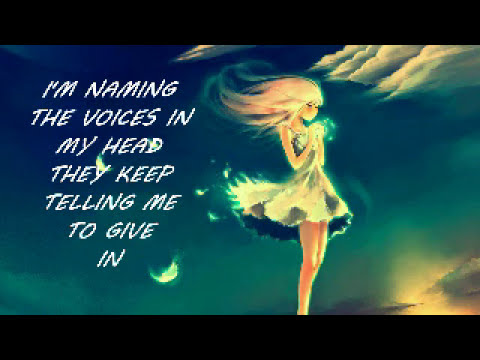The digital image is a highly detailed piece of pixel art featuring a fairy-like girl with a magical aura. She has flowing white and pink hair, blown whimsically upwards, and she's adorned in a short, airy dress that billows behind her, with feathers seemingly floating off into the sky. The character appears to have a light skin tone and exhibits a delicate, ethereal quality, as she faces to the left, hands clasped in front of her. Her downward gaze is accentuated by dark eye lines, hinting at an Asian appearance. She's surrounded by a dark blue sky sprinkled with wisps of clouds, blending into a subtle sunset in the top right corner. Near her hands, she's conjuring something magical, illuminated by blue, swirling stars. The composition is bordered by horizontal black bars. The left side of the image features white pixelated text that reads, "I'm naming the voices in my head, they keep telling me to give in." This adds a contemplative, almost melancholic dimension to the scene, enhancing the mystical and otherworldly atmosphere of the artwork.